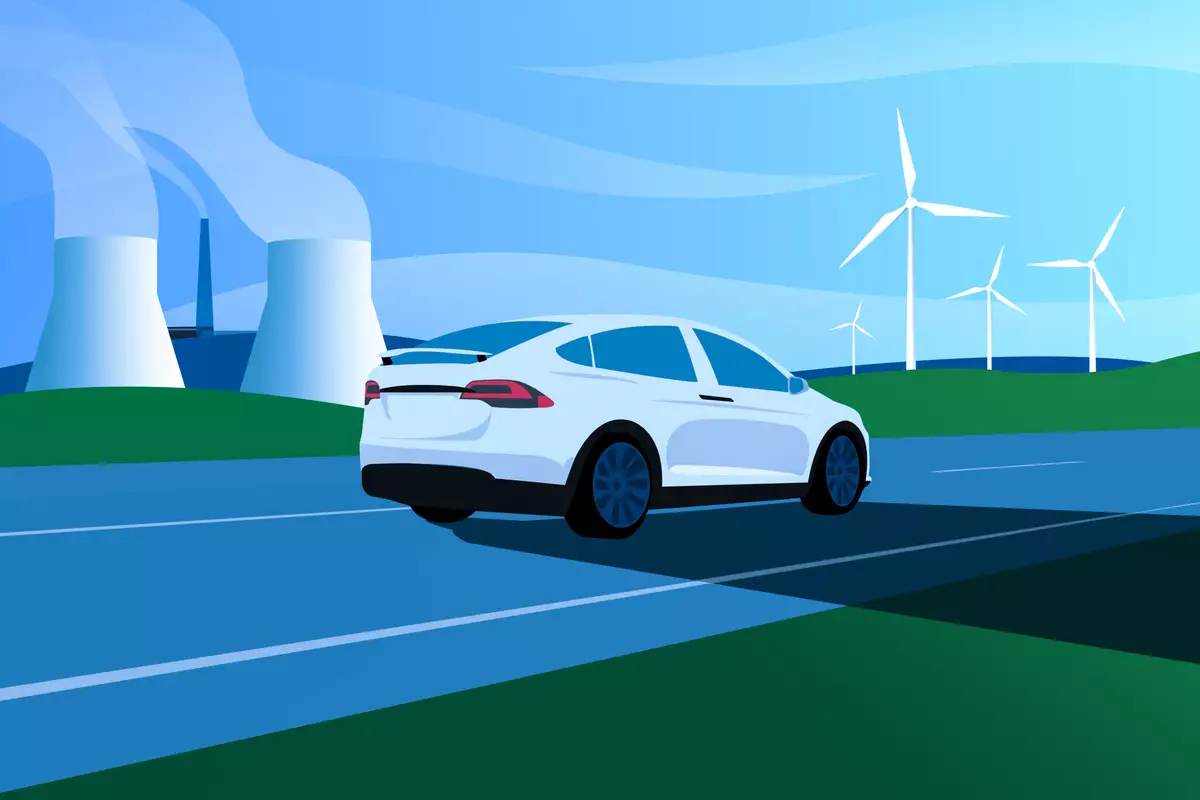The digital illustration portrays a white car driving along a blue road, bordered by green fields. The car, featuring blue rims, blue-tinted windows, and red taillights, navigates on the right side and may be a coupe due to its single visible door. In the background, the scene is split between two contrasting landscapes. To the left, under a darkened sky, two or three nuclear power plants emit white steam. On the right, against a lighter, swirling blue sky, a wind farm with four white wind turbines stands amid the green fields. The car casts a shadow away from the nuclear power plants, symbolizing its movement towards the wind farm. This striking composition, created with flat colors and digital artistry, suggests a narrative contrast between older and renewable energy sources.